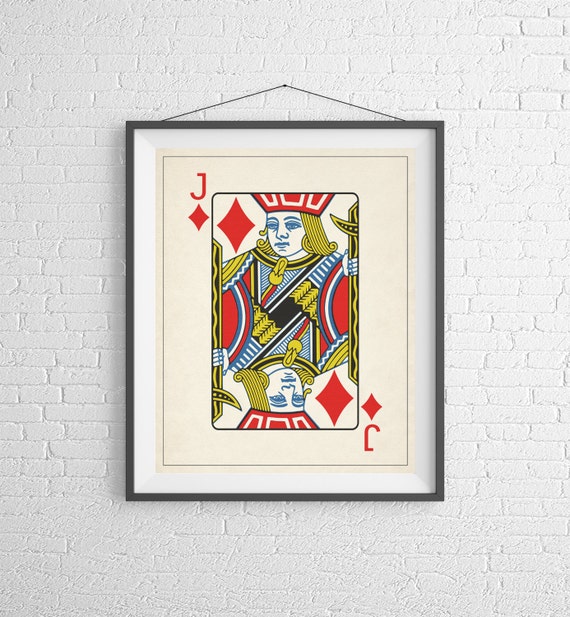The image depicts a photograph of a framed painting of a red Jack of Diamonds playing card, centrally positioned against a white brick wall. The painting is encased in a thin black vertical rectangular frame, bordered by white on all sides. The red Jack of Diamonds card inside the frame features a detailed portrayal of the Jack, adorned with a red crown and traditional royal attire. The card exhibits a mirrored image, with the Jack's face and upper body oriented normally at the top and mirrored at the bottom. In the top left corner of the card, a large red diamond and a smaller red diamond can be seen next to the letter "J". Similarly, in the bottom right corner, there is a mirrored "J" alongside a large and small red diamond. The frame is suspended by a thin black wire or thread, stretching diagonally upwards toward a small nail or tack, securing it to the wall.